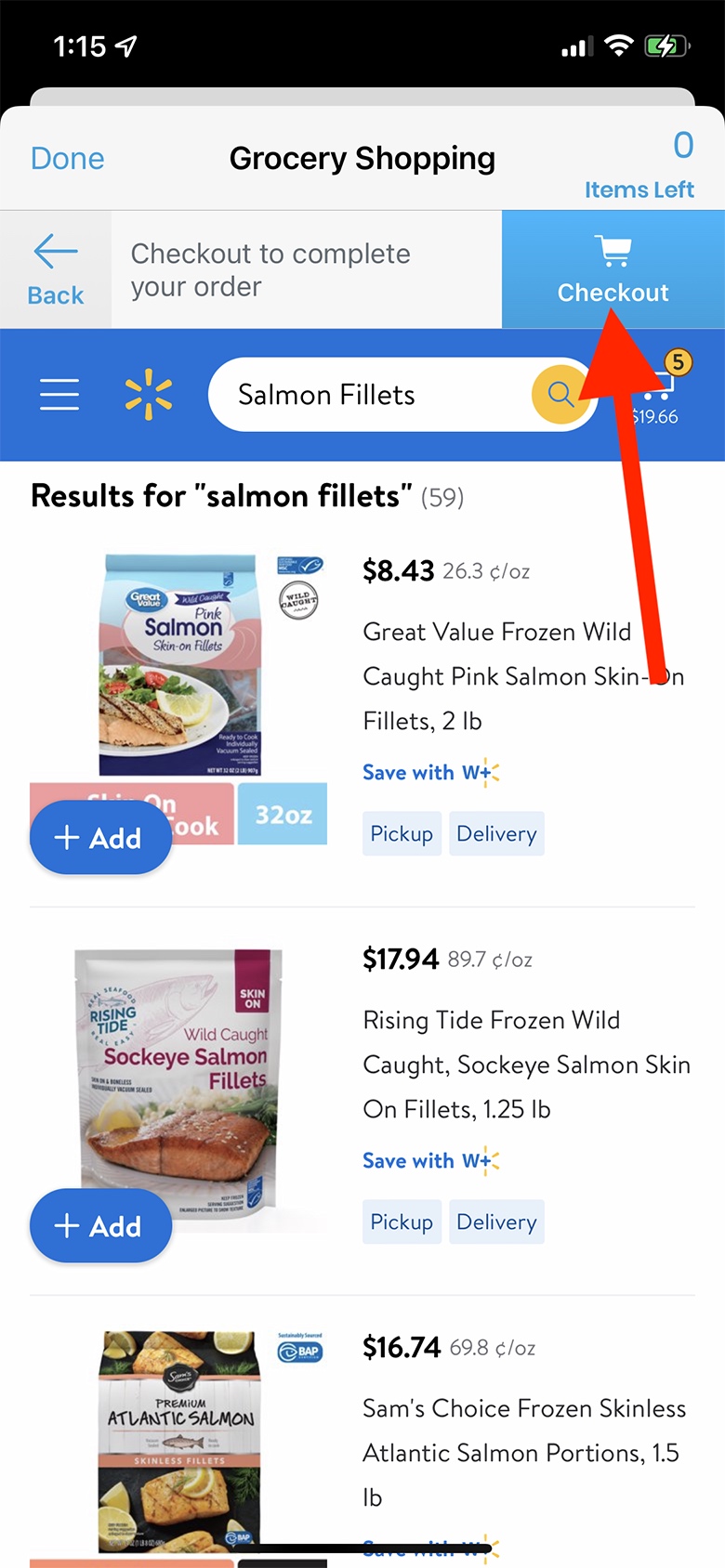Screenshot of Walmart Grocery Shopping Search Result for Salmon Fillets:

The image is a screenshot from the Walmart website featuring grocery shopping search results. At the top, the page is titled “Grocery Shopping.” On the right side of the screen, a prominent red arrow points directly to the "Checkout" tab, guiding the viewer's attention there. 

Below the navigation bar, the search box shows the term "salmon fillets," indicating that the user has searched for this item. The search results display a variety of salmon fillet options, with detailed listings. Notable among these is an $8.43 option for "Great Value Frozen Pink Salmon, Skin-On Fillets" weighing 2 pounds. Another highlighted option is the $17.94 "Sockeye Salmon, Skin-On Fillets." This detailed information is clearly presented, making it easy for the viewer to compare the different brands and prices of salmon fillets available for purchase on Walmart's grocery shopping platform.